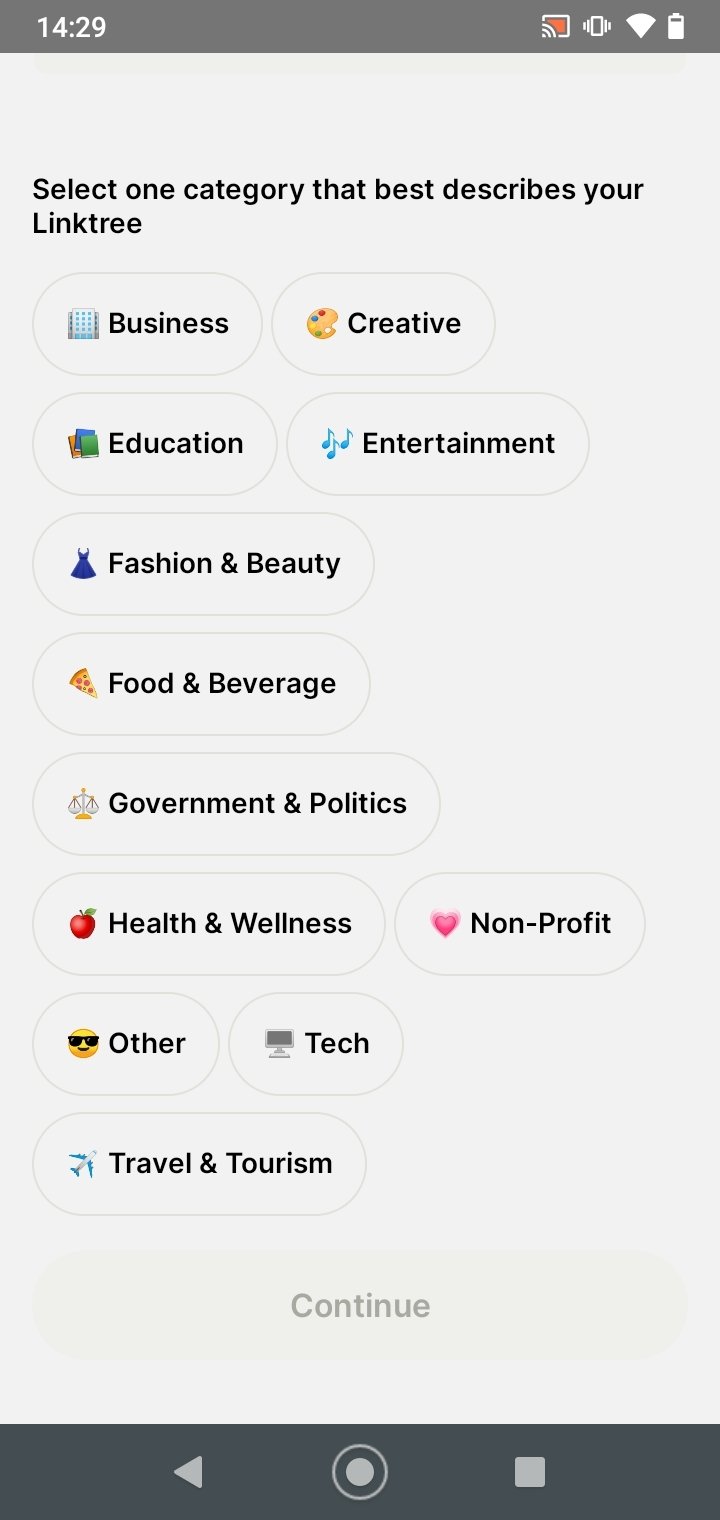The image is a cell phone screenshot. At the top is a grey dotted line. In white text on the left, the time is displayed as 14:29, indicating 2:29 PM. On the right side of the screen, there are icons showing a cell phone with screen sharing enabled, a vibrate mode indicator, full Wi-Fi signal strength, and approximately 75% battery remaining.

Below this, on a grey background with black text, there is a prompt: "Select the one category that satisfies your weak tree." The following categories are listed:
- Business
- Creative
- Education
- Entertainment
- Fashion and Beauty
- Food and Beverage
- Government and Politics
- Health and Wellness
- Non-Profit
- Other Tech
- Travel and Tourism

At the bottom of the screen, there is a greyish button labeled "Continue." The phone’s navigation bar features a back arrow on the left, a home button in the middle, and a square (likely for recent apps) on the right, all against a grey-black background.

The image captures a moment frozen in time, meticulously detailing the interface and various UI elements of the cell phone screen.